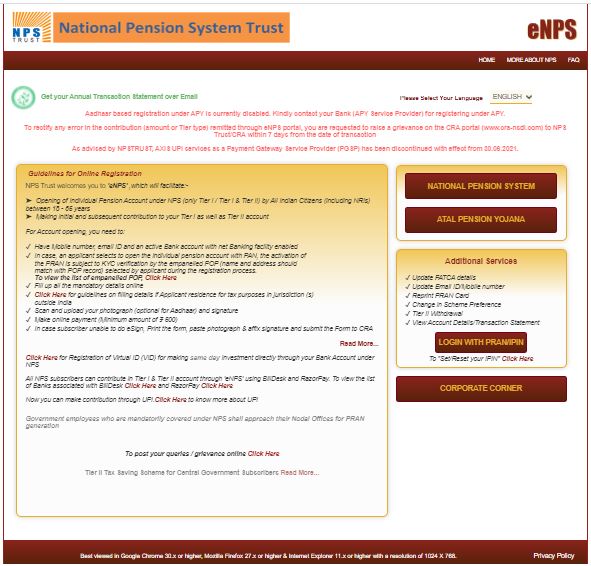This image depicts a web page from the National Pension System (NPS) Trust, primarily featuring a white background. 

At the top left corner, you will see the acronym "NPS" displayed prominently in bright blue letters. Directly beneath it, the word "Trust" appears in grey letters. Adjacent to this, there is a distinctive logo resembling rays of light, or orange lines, emanating from the term "NPS Trust," symbolizing rays of sunshine. 

To the right of this logo, an orange rectangular horizontal box includes the text "National Pension System Trust" in blue letters. Furthest to the right on the same line, the term "eNPS" is written in a dark brown font, with a lowercase "e" followed by uppercase "NPS."

Below these elements, a thin, dark chocolate brown ribbon traverses the width of the page. On the right end of this ribbon, white text denotes menu options, including "Home" and "More About Us." 

Beneath this ribbon, on a white background, there is a small section of bright blue text reading "Get your annual transaction statement over email." This prompt is accompanied by a turquoise circle with a logo inside. To the right of this, there is a prompt for language selection, currently set to English, with an adjacent dropdown menu.

Further down the page, there is a block of four lines of bright, dark pink text, though the text is too small to read clearly. Below this, a large rectangular box is bordered by a thin grey line, containing extensive black text. 

To the right of this large box, two additional smaller boxes with thin borders are displayed. The first of these contains two dark brown buttons. One button is labeled "National Pension System" in gold, and the other is labeled "Pension." The second box, situated below the first, is marked "Additional Services."

The page's design incorporates a structured layout with organized sections, clearly demarcated by colors and borders, ensuring user-friendly navigation for visitors seeking information related to the National Pension System Trust.